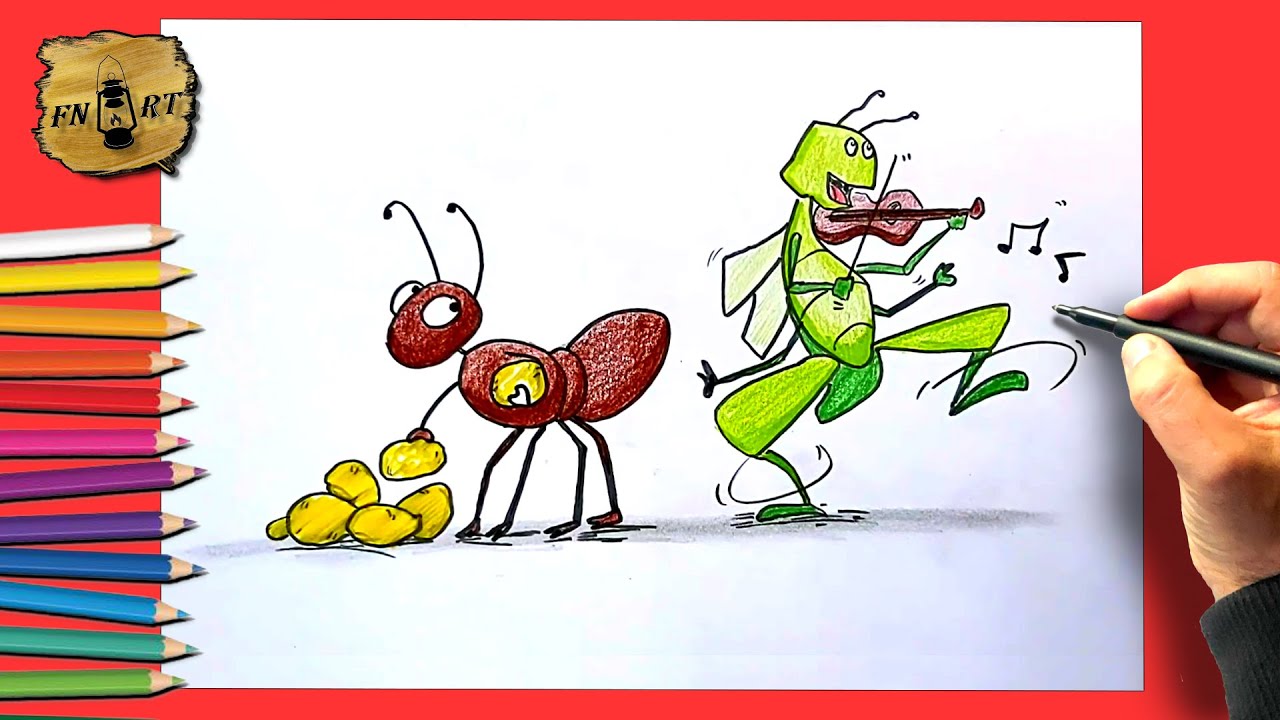This image is a horizontally rectangular cartoon illustration, approximately six inches wide and three inches high, resembling an advertisement. It is framed by a thin red border at the top and bottom, and a thicker red border on the left and right sides. In the upper left corner, a wooden cutout with a lantern logo and the text "FN Art"—where the lantern forms the letter "A"—is displayed. Below this logo are twelve sharpened, multicolored pencils in a progression from white, yellow, light orange, dark orange, reddish-orange, pink, purple, dark purple, blue, light blue, greenish blue, to green.

On the right side of the image, a light-skinned hand with a gray sleeve is seen holding a black marker, drawing on a white sheet of paper. The paper features a cartoon depiction of two insects: a red ant and a green grasshopper. The ant, located on the left, is gathering yellow circular objects from the ground, which might be food or crumbs. Its body is turned away from the grasshopper but its eyes are looking towards it, indicating curiosity or confusion. The green grasshopper on the right is animatedly playing a brown violin or fiddle, with one leg kicked up and music notes surrounding it, suggesting it's dancing. The backdrop of the entire illustration is a rich red color.